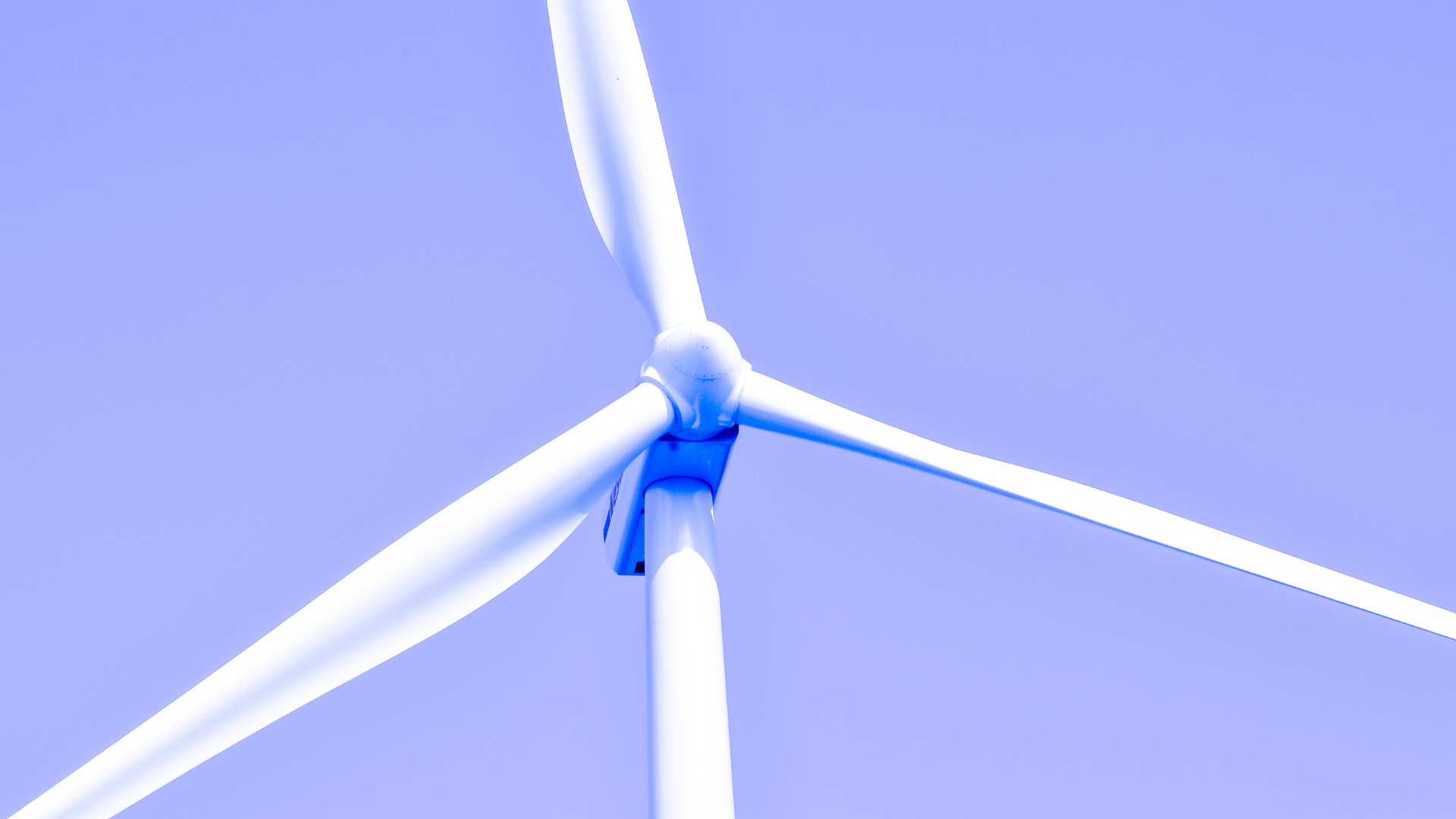The image showcases a close-up of the upper section of a modern wind turbine set against a bright, clear blue sky. The turbine's white blades are prominently displayed, although their tips extend beyond the edges of the image, emphasizing their considerable length. At the center, the hub, which appears slightly bluish likely due to reflections and shadows, connects the three blades to the white post. One blade points directly upward, while the other two angle downward diagonally to the left and right. The image is devoid of any other objects or details, contributing to a serene and isolated visual effect. The wind turbine itself appears stationary, enhancing the static and peaceful ambiance of the scene.